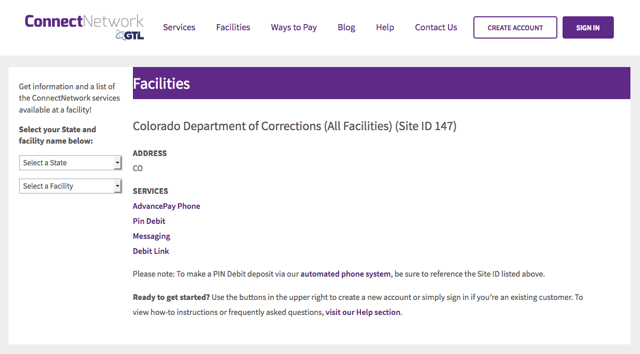The image depicts the Connect Network GTL website, featuring a predominantly purple-themed design except for two lines on the left and the right where the address and services are printed in black. At the top, there's a horizontal purple bar with the word "Facilities" written in white, serving as a navigation tab. 

On the left side of the page, there is a column titled "Get Information" that lists the available Connect Network services for different facilities, with dropdown options to select your state and specific facility. The section currently viewed is for the Colorado Department of Corrections, encompassing all its facilities. The Site ID for this specific section is 147. 

The address is specified as Colorado, and the services available include Advanced Pay Phone, Pin Debit, Messaging, and Debit Link. A notable instruction states that to make a Pin Debit deposit via the automated phone system, users must reference the listed Site ID. The page concludes with a prompt: "Ready to get started."